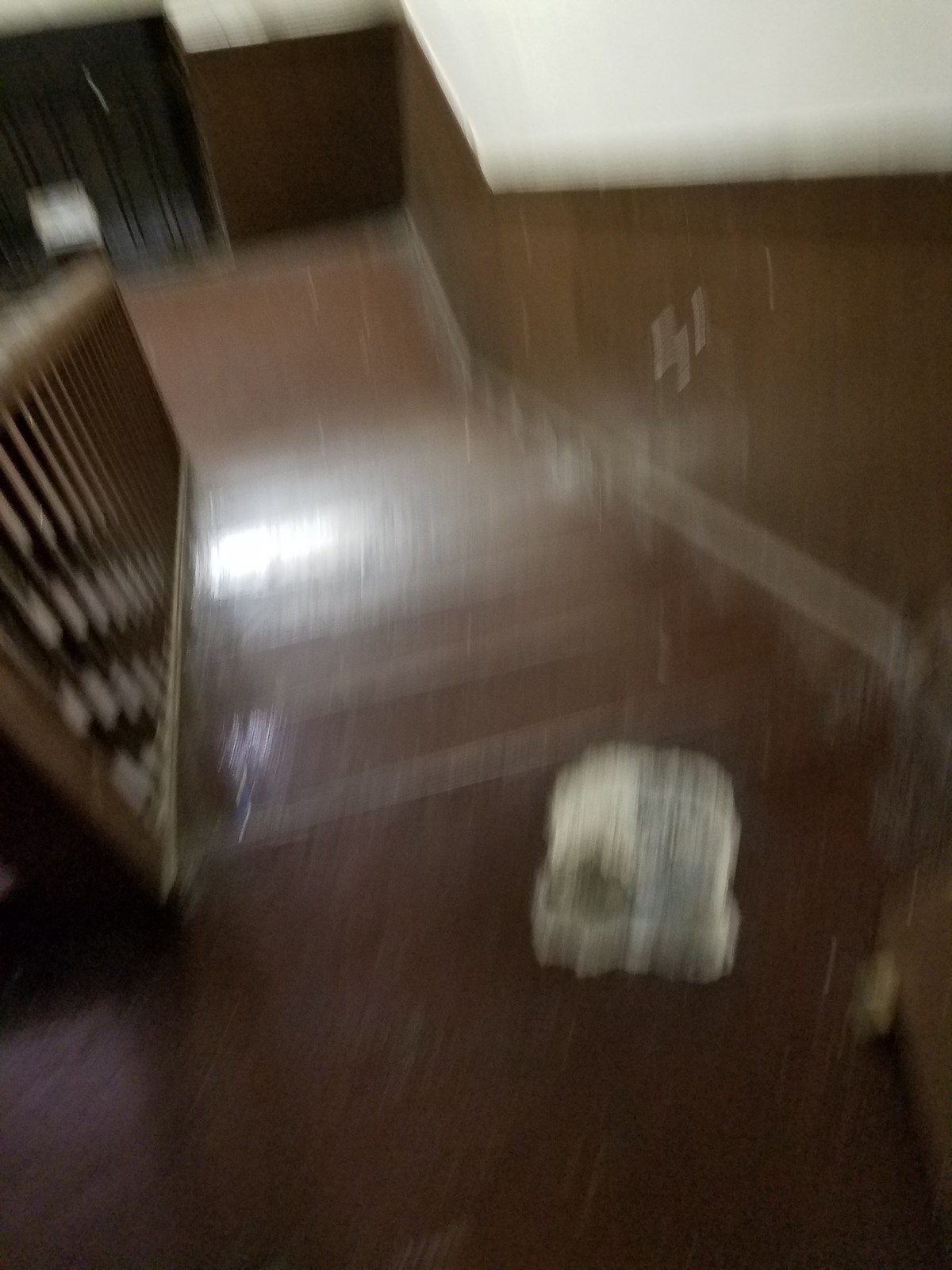The image depicts a very blurry interior view of a staircase taken from a landing area. It is vertically rectangular and the vantage point appears to be from the top of the stairs, looking downward. The staircase is framed by white walls that extend from the top portion of the frame, transitioning to a dark brown wood grain on the lower half. The landing, steps, and floor at the bottom share this dark brown wood grain, creating a consistent, rich hue throughout the scene.

A hand railing with vertical decorative dowels is visible to the left side of the stairs. Notably, affixed to one of the walls, there is a number '41,' though it's also blurred. At the bottom right portion of the image, there is a blurred, white square object with some black markings, which may suggest a pile of newspapers awaiting distribution, likely in what seems to be an apartment building. Additionally, patches of sunlight create sunspots that dot the stairs and parts of the image, illuminating sections of the wooden surfaces and a black door visible at the bottom of the stairs. The mixture of brown and white elements accentuates the contrast between the dark, rich wood and the bright, sunlit areas.